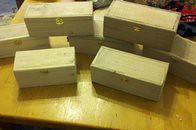The low-resolution image features a close-up of a pine wood table, showcasing its grain texture. Atop the table, there are seven long, rectangular wooden boxes, similar in appearance to those used for storing cigars. These boxes are a pine wood color and are each secured with a small metal latch on the front. The arrangement consists of two boxes placed side by side in the foreground, with the remaining five boxes forming a pyramid-like stack behind them—three on the bottom and two on top. The setup casts noticeable shadows on the table due to a light source from above. The background, hinting at a home environment, appears to be a white floor.